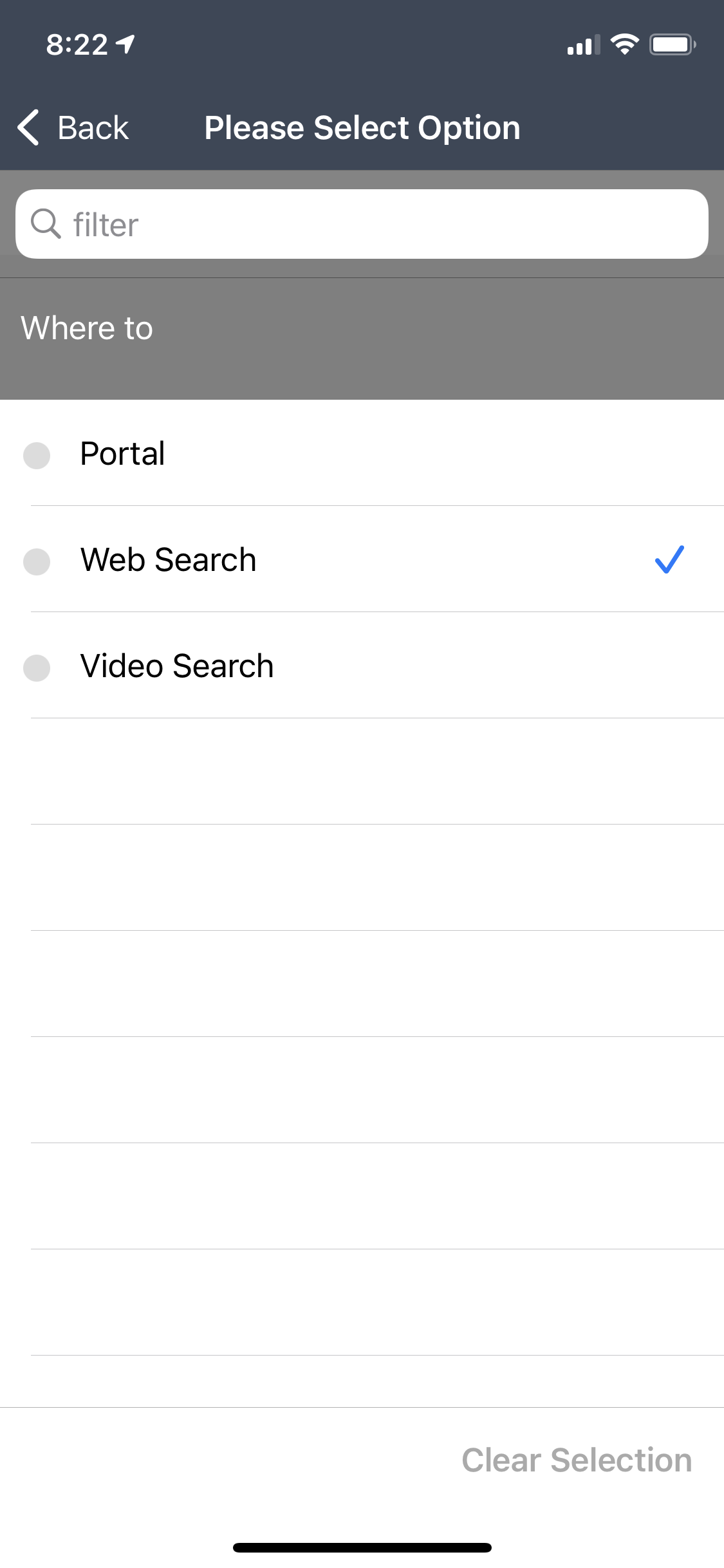Screenshot of a cell phone displaying a "Please Select Option" screen:

The overall background is predominantly white. At the very top, a black bar spans horizontally, containing white text and icons. On the far left, the current time reads "8:22," accompanied by an upward-right arrow. To the far right, there are three connectivity bars, a Wi-Fi icon, and a battery level indicator.

Below this top bar, from left to right, are navigation elements: a left-pointing directional arrow, a "back" button, and the text "Please Select Option." Below this, a gray rectangular area prominently features a horizontal, white search bar at its top. The search bar includes a light gray magnifying glass icon and a filter icon.

Inside the gray rectangle, beneath the search bar in white text, it reads "Where to?" Underneath this text, there are three vertically stacked gray dots, each accompanied by a word. The first dot, labeled "Portal" in black text, is followed by a thin gray line running horizontally. The second dot, labeled "Web Search," is marked with a blue check icon to its right. Another horizontal gray line follows below this option. The third and final dot, labeled "Video Search," is in black text.